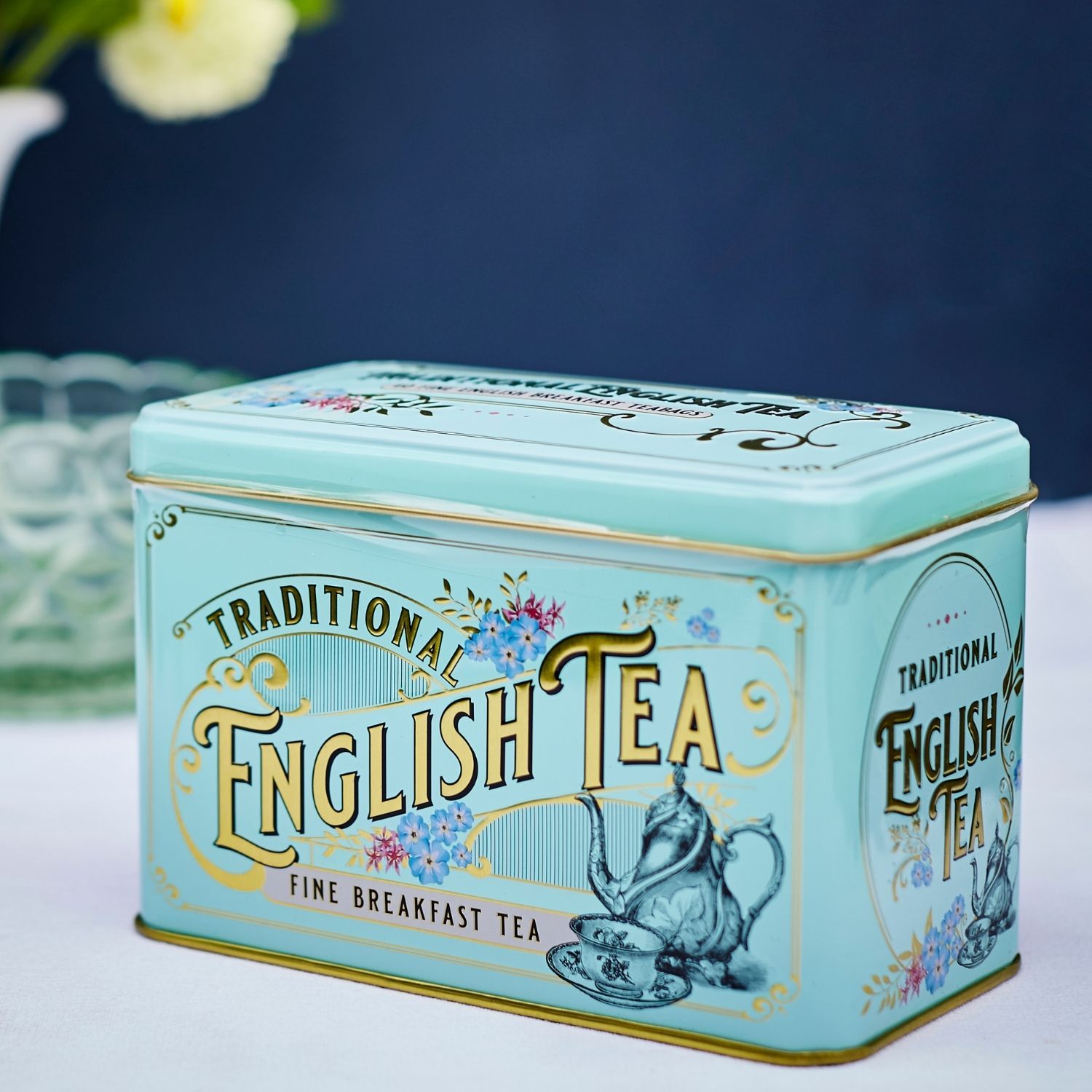This detailed close-up photograph features a sophisticated light powder blue metal tea tin with a rectangular prism shape and gold trim. On the front, the elegant gold inscription reads "Traditional English Tea," with a small pink and black label below stating "Fine Breakfast Tea." The tin showcases a charming old-fashioned teapot with a floral design, accompanied by a matching fancy teacup and saucer. The entire tin is adorned with delicate floral patterns, including blue and pink flowers with green leaves. The tin's lid is visible, though partially obscured, and the container is angled slightly to the left, allowing a partial view of its side and top.

In the blurred background, there is a dark navy blue wall, a clear crystal decorative bowl, and a white vase. A hint of a daffodil with a green stem and white petals with a yellow center peaks out from the vase. The surface on which the tin rests is a light gray counter, providing a subtle contrast to the tin's blue shade.